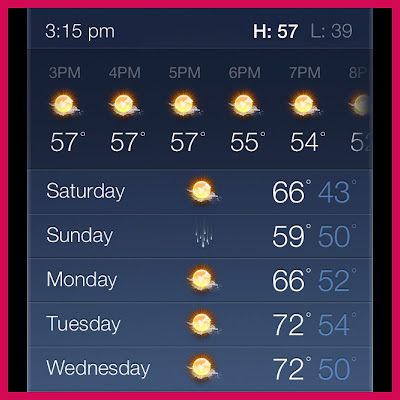The image is a screenshot displaying a weather forecast at 3:15 PM. The highlighted 'high' temperature is 57°F, with a 'low' of 39°F. The top section shows an hourly breakdown from 3 PM to 8 PM, indicating sunny conditions with scattered small clouds throughout. The temperatures are 57°F at 3 PM, 4 PM, and 5 PM, then dip slightly to 55°F at 6 PM, 54°F at 7 PM, and approximately 52°F at 8 PM, which is partially cut off.

The forecast also includes icons indicating weather conditions, with mostly sun and some clouds for each hour. The extended forecast covers Saturday through Wednesday, predicting daily highs of 66°F, 59°F, 66°F, 72°F, and 72°F, respectively, with nightly lows predominantly in the 50s, except for Saturday night, which will dip to 43°F. Additionally, Sunday shows a chance of precipitation, while other days remain mostly sunny with minimal cloud cover.